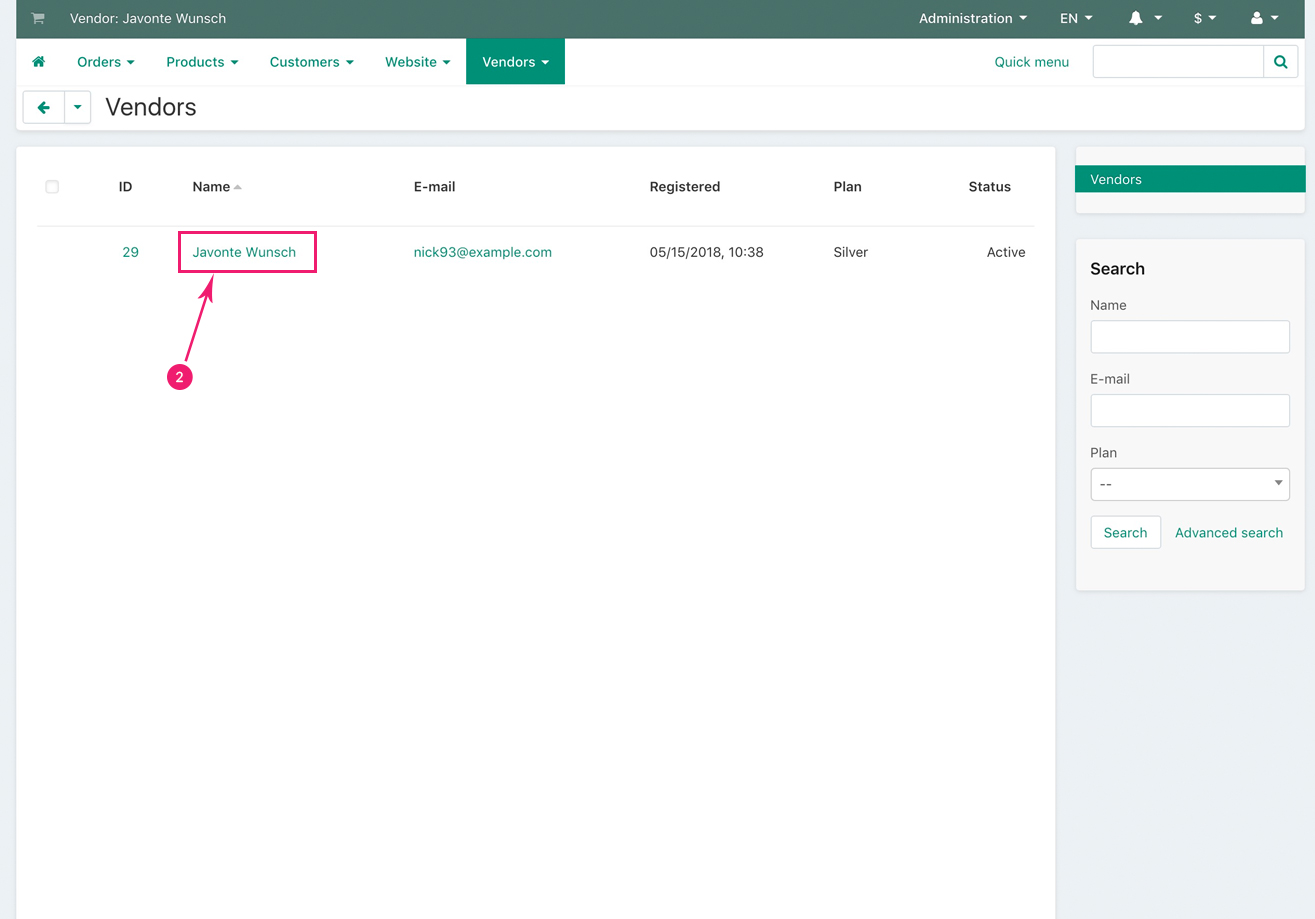This image is a detailed screenshot from the vendor management section of a business management software platform. The interface is sleek and well-organized, featuring tabs for orders, products, customers, website, and vendors at the top, indicative of a comprehensive system for managing various business operations.

The highlighted section in the image is the 'vendors' tab, showcasing a list of various vendors. The main content area is organized into columns for ID, Name, Email, Registered Date, Plan, and Status. 

Currently, the details of one specific vendor are listed:
- **ID:** 29
- **Name:** Jovante Wunsch
- **Email:** nick93@example.com (a placeholder email)
- **Registered Date:** 05/15/2018 at 10:38 (AM/PM not specified)
- **Plan:** Silver
- **Status:** Active

The vendor's name, Jovante Wunsch, is highlighted and pointed to by a pink arrow, indicating that it is currently being edited or is the focal point of attention in this section.